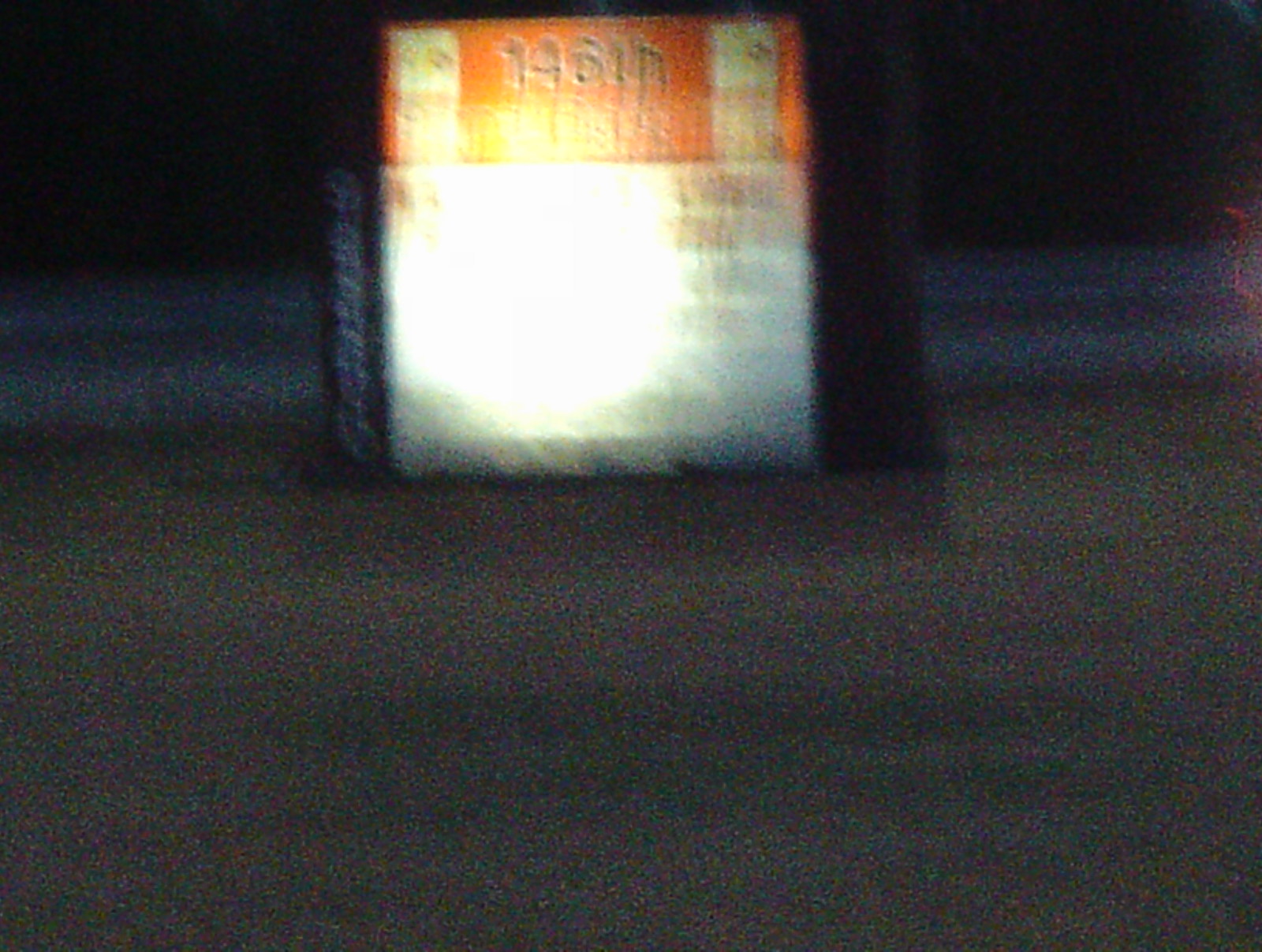The image depicts a blurry and dark scene, possibly at night, with a greyish, grainy surface below and darker hues, including black and blurry dark blue, above. The midsection of the image features an illuminated object, potentially a thick sign or a box, with the numbers "146" prominently displayed on it. The bright light from behind this object is so intense that it obscures much of the surrounding details, making it nearly impossible to discern specifics. There appears to be a metal surface nearby, possibly reflecting the artificial light. Additionally, there are hints of vertical black bars on either side of the illuminated object. In the background, the image grows even darker, with the suggestion of a guardrail, typical of those seen on interstates, and potentially some red thread on the right side near the guardrail. Overall, the image is very blurry, making it difficult to identify precise elements, but the combination of these observations suggests an ambiguous and intensely lit scene with minimal visibility into the deeper background.